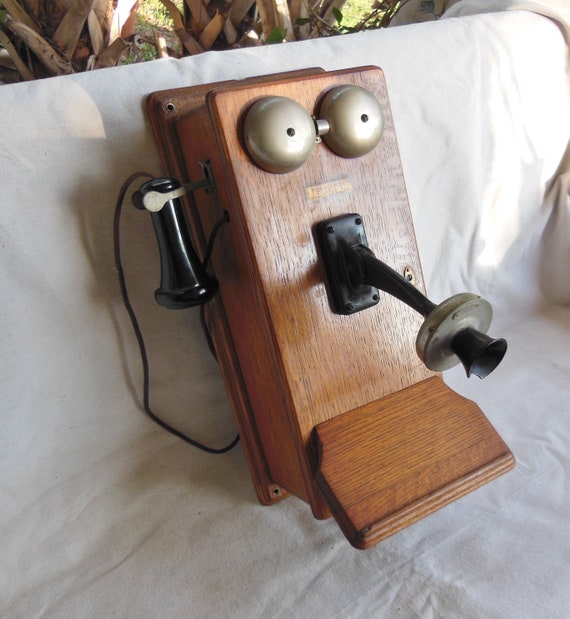This image features a classic wooden telephone from the 1930s or 1940s, prominently positioned in the center of the frame. The backdrop appears to be an outdoor setting with palm trees visible, hinting that the photo was taken outside. The telephone, crafted from brown wood with metal and black components, is propped up against a white sheet that seems to be draped over a seating arrangement, possibly a loveseat. The device itself includes two round gold bells at the top, a black cylindrical ear speaker hanging on a cord, and a long microphone fixed to the front. The subtle copper hues add a touch of vintage charm to this old-fashioned communication device.